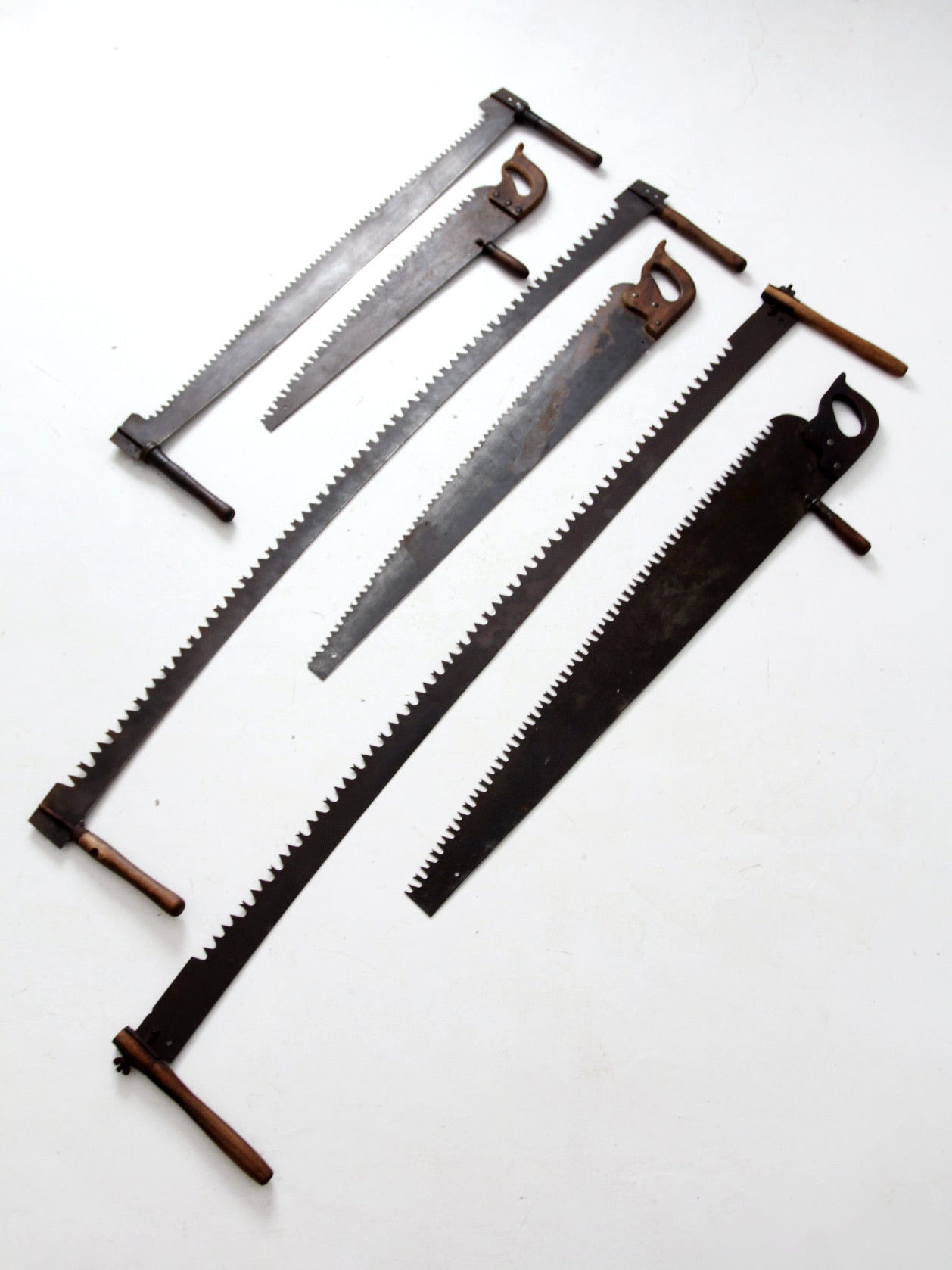This color photograph captures six vintage saws arranged diagonally from the top left to the bottom right against a white, slightly shiny background. The saws, which exhibit a well-used patina indicating their age, are laid out in an organized, parallel manner, starting with the smallest and ending with the largest.

The saws are divided into two categories: three two-person saws and three one-person saws. The two-person saws, featuring handles at both ends, include a small, a medium, and a large variant. These saws have long, slender blades designed for tandem use, often in logging, with the smallest saw at the top left having a straight blade, the medium saw with a gentle arch, and the largest being the most substantial in size.

Interspersed between these are three one-person saws. The smallest one-person saw follows the first two-person saw and is of a traditional design with a single handle. The next one-person saw, positioned after the medium two-person saw, has an additional top handle on the back of the blade for extra control. The largest one-person saw, placed after the largest two-person saw, also features a dual-handle design for enhanced stability during use.

Overall, the saws form a symmetrical and graduated pattern, providing a comprehensive look at these antique woodworking tools under a bright overhead light that emphasizes the metallic surfaces and fine details of the blades and handles.